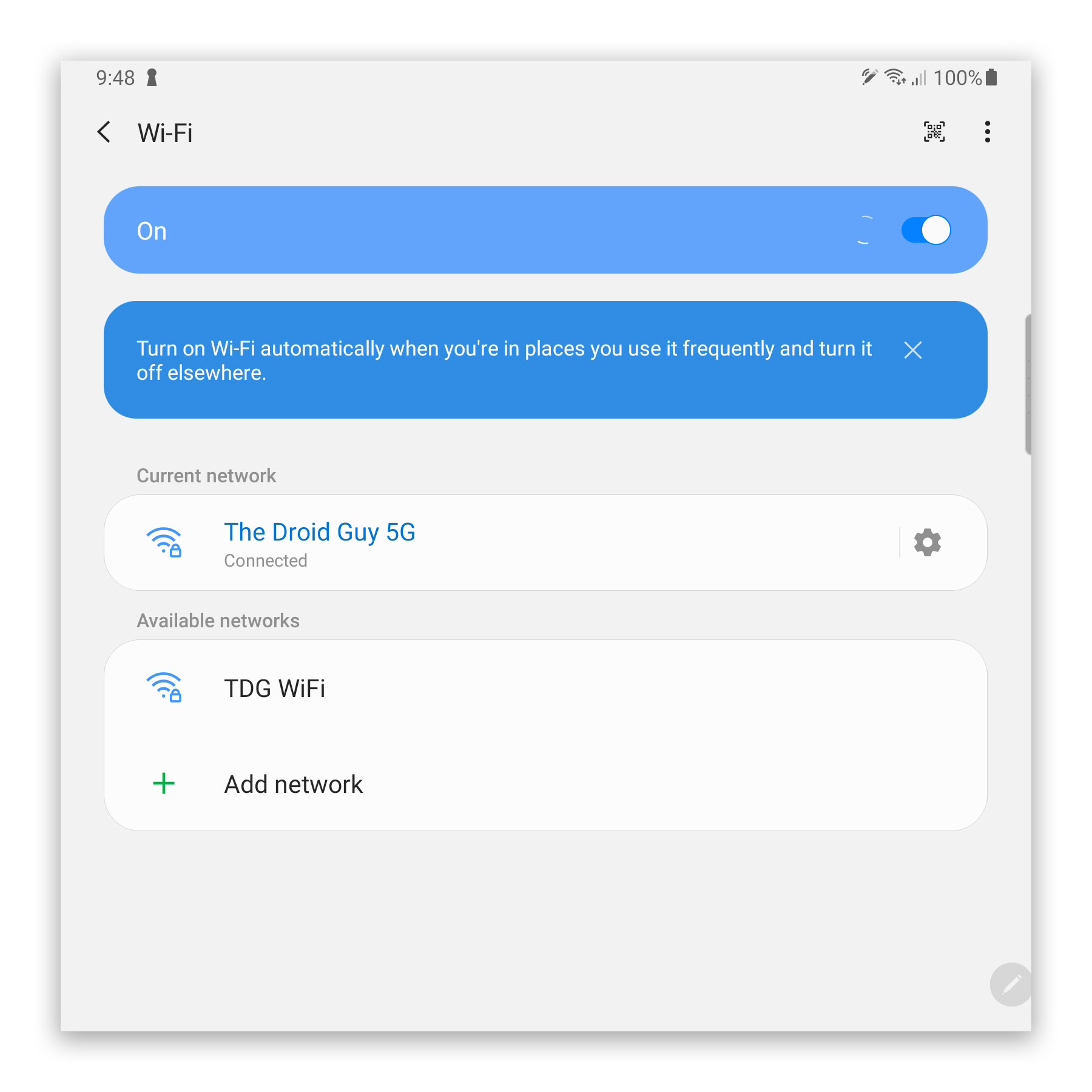The image displays a screen capture of a smartphone interface set against a slightly off-white background. In the top-left corner, the time is displayed as "9:48" in black text. Adjacent to this, there is a keyhole icon. On the right-hand side, the status bar showcases several indicators: a Wi-Fi signal with two bars, a cell signal icon with two out of four bars filled, the text "100%" in light gray, and a fully charged battery icon in dark gray.

Beneath the status bar, on a white background, there is a black left arrow followed by the text "Wi-Fi" in large letters. On the far right, close to the edge, there are an "X" symbol and three vertical dots arranged in a column.

Below the "Wi-Fi" header, there are two blue oval buttons with white text. The first button reads "ON," and to its right, an on-off switch with a white dot is slid to the "on" position. The second button states, "Turn on Wi-Fi automatically when you're in places you use it frequently and turn it off elsewhere."

The next section is labeled "Current Network" in black text. Within this section, there are two oval areas on a white background. On the left, a blue Wi-Fi signal icon and blue text indicate the network name "SIDROID GUY 5G," with the status "Connected" written in black beneath it. To the right of this, a gray settings gear icon is visible.

Following this, the section "Available Networks" is displayed in black text. Within this section, a white background displays another Wi-Fi signal icon followed by the text "TDG Wi-Fi" in black. Below this, there is a blue "Add Network" button.